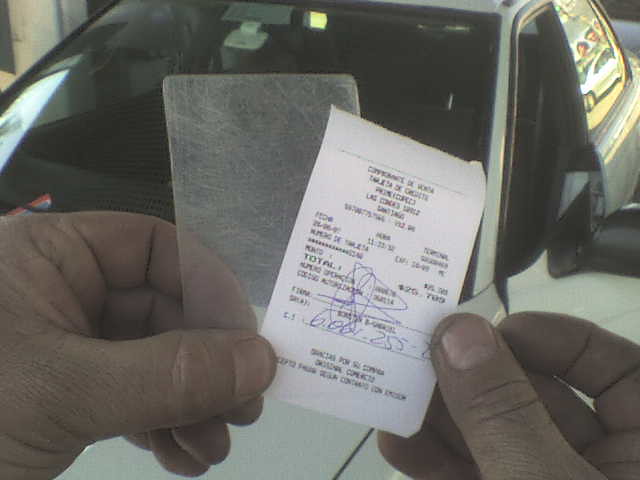In this photograph, a pair of hands holds up a white, partially legible receipt, which is possibly written in Spanish, and another similar-sized piece of paper, spread out like cards. The receipt appears to have a substantial amount, possibly around twenty-six thousand dollars, and includes a signature and some numbers at the bottom, written with a blue pen. The scene is outdoors, likely under a carport. In the blurred background stands a white car with an open front door, revealing the windshield, front driver's side door, rearview mirror, and partially visible roof and back window. The photo captures the receipt held between the thumbs and index fingers, with the fingertips of both hands visible.